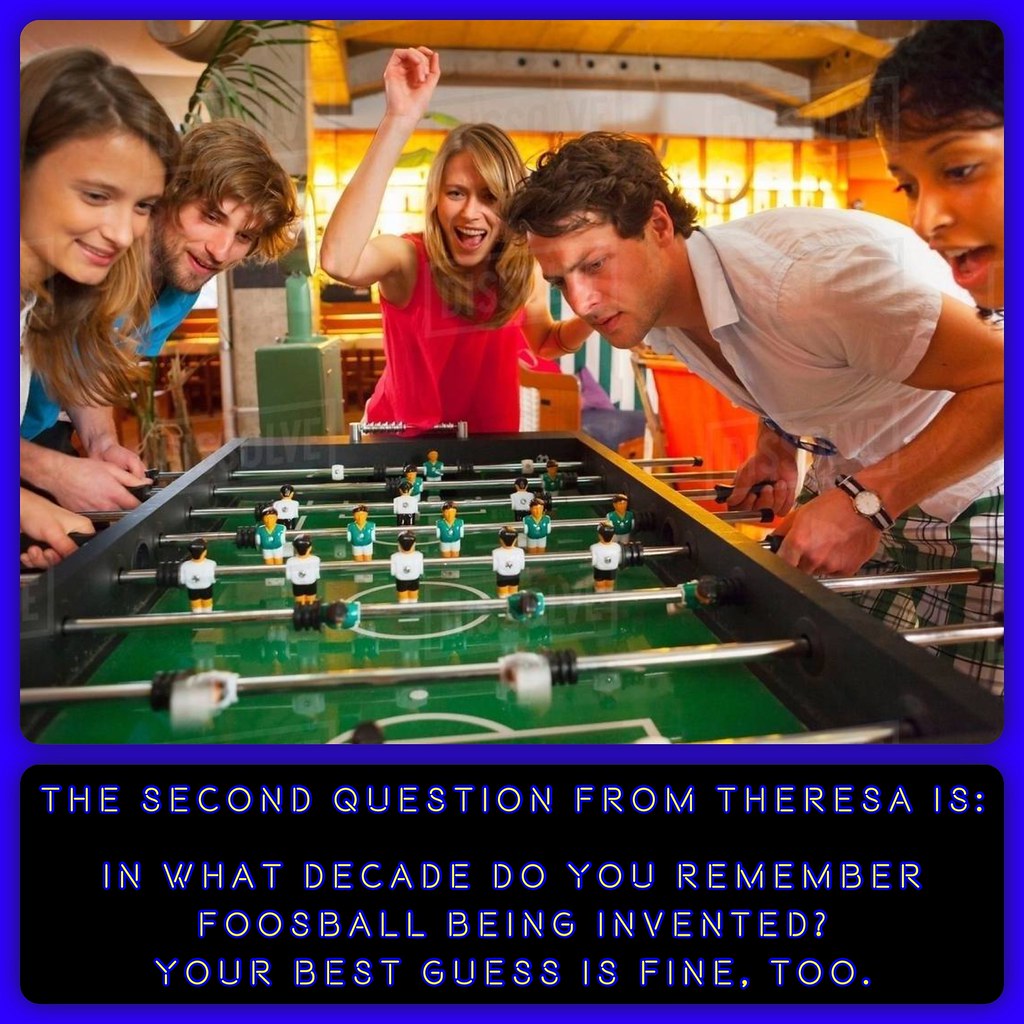This vibrant, color photograph captures a lively foosball game in progress, framed within a landscape orientation but altered to a square format through added typography and graphic design elements. The image is divided into a top portion featuring the action and a bottom black horizontal panel with white text that reads: "THE SECOND QUESTION FROM TERESA IS: IN WHAT DECADE DO YOU REMEMBER FOOSBALL BEING INVENTED? YOUR BEST GUESS IS FINE, TOO." 

The top two-thirds of the image showcase a foosball table with a green playing field. The two teams are distinguishable by their attire: one team wears green shirts and white pants, while the other dons white shirts and black pants. Players and onlookers are clearly engaged in the game. To the left, there's a young woman, seemingly in her early twenties, partially cut off by the frame. Beside her stands a man with long hair and a beard, wearing a blue shirt. At the end of the table, a woman in a red shirt, with brown hair cascading over her shoulders, laughs with her right hand raised. On the right side, a mid-20s man in a white shirt leans over the table, focusing intently on the game. Beside him, an African-American woman in her twenties, mostly visible through her hair, eyes, and mouth, also concentrates on the game. A hint of green plaid pants can be seen on another individual near her.

The background is illuminated with soft yellow lights, suggesting an indoor setting with a counter. The entire image is bordered by a dark blue frame, enhancing its visual appeal while integrating the typographic question from Teresa, making it both an engaging and informative piece.